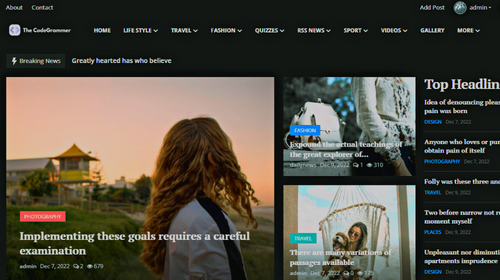Screenshot of a website with a black background. In the upper left corner, the navigation options "About" and "Contact" are displayed in white letters. On the upper right corner, there are "Add Post" and "Admin," with a dropdown arrow next to "Admin." The header includes site navigation items: starting from the left, "Home", "Lifestyle" (with a dropdown menu), "Travel" (with a dropdown menu), "Fashion" (with a dropdown menu), "Quizzes" (with a dropdown menu), "RSS News" (with a dropdown menu), "Sports" (with a dropdown menu), "Videos" (with a dropdown menu), "Gallery", and "More" (with a dropdown menu).

Below the navigation bar, there's a "Breaking News" section. Next to it, phrases such as "greatly hearted," "has who," and "relieve" are visible, although their context is unclear. The main content area features a prominently displayed photograph of a girl with long blonde hair, facing away from the camera and wearing a white or light blue shirt. The caption accompanying the image reads, "Implementing these goals requires a careful examination," attributed to Admin, dated December 7, 2022. An orange-pink button labeled "Photography" sits below the caption. The background shows a beach house on stilts during a picturesque sunset or sunrise.